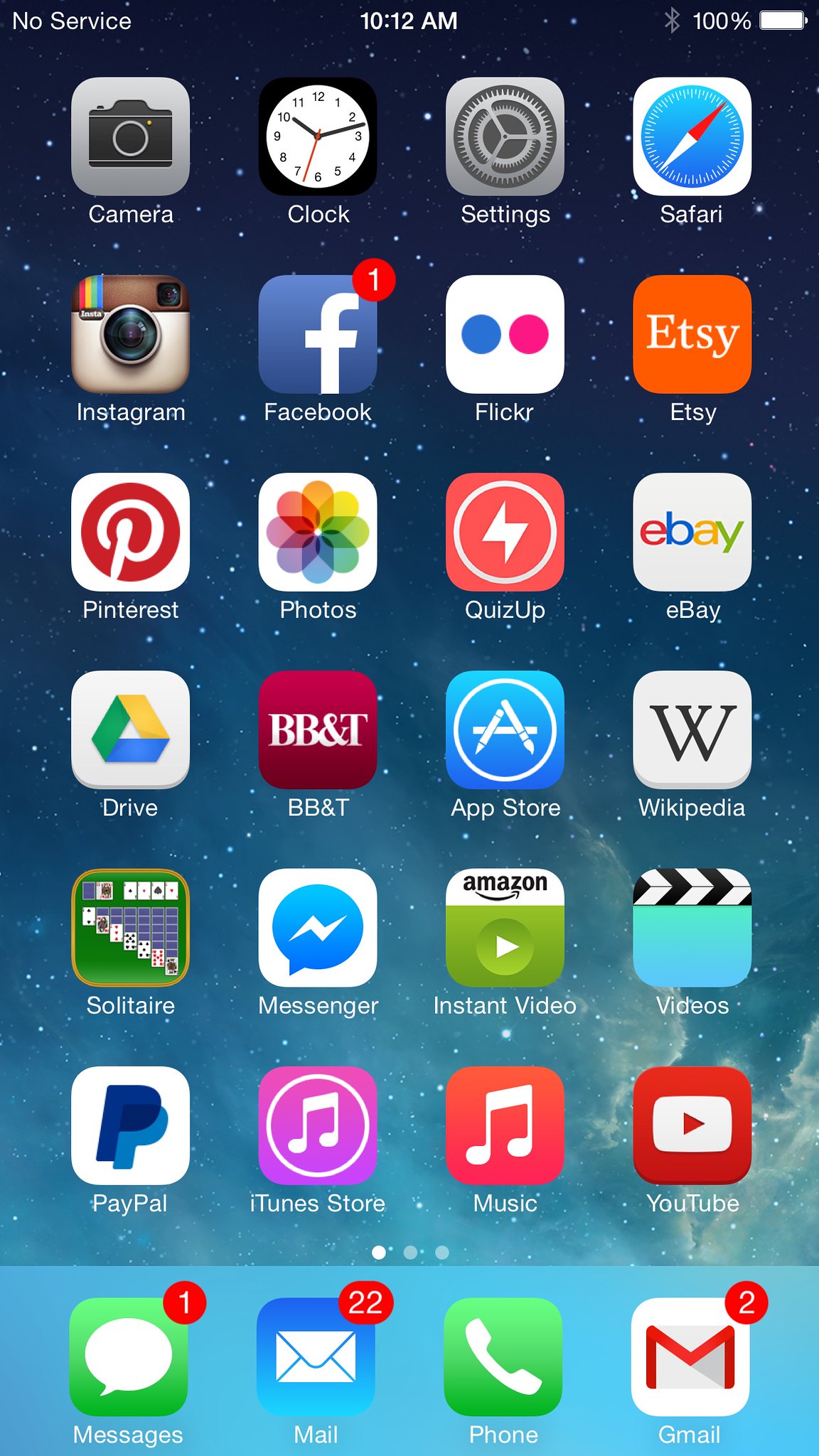A detailed descriptive caption for the described image:

---

The image captures a screenshot of a smartphone's home screen, presented in a vertical orientation with a starry background. At the top left corner, the status bar displays "No Service" in a small white font, indicating that the phone has no cellular connectivity. Centrally positioned in the upper section, the time is shown as 10:12 AM. Adjacent to the time, the Bluetooth icon is visible, followed by a battery status indicating the phone is fully charged at 100%.

The home screen shows a 4x6 grid of app icons with four additional shortcuts pinned to the dock at the bottom. The dock's background is a slightly lighter blue compared to the starry theme of the main screen. The following details are observed:

- **Messages**: A red circular notification badge with a white "1" in the upper right corner, denoting one unread message.
- **Mail**: Exhibiting a red badge with a white "22," indicating twenty-two unread emails.
- **Phone**: No notification badge present.
- **Gmail**: A red badge with a white "2," marking two unread emails.

Among the 24 app icons on the main screen, recognizable ones include the Camera, Clock, Settings, and Safari. Notably, Facebook appears on the second row with a red notification badge illustrating one unread notification. An unusual icon labeled "Quiz Up" is located on the third row. Additionally, the screen displays icons for BB&T, likely a financial application, and Solitaire, a game app.

---

This caption provides a comprehensive and structured description of the smartphone home screen, highlighting key details and notifications present on the device.